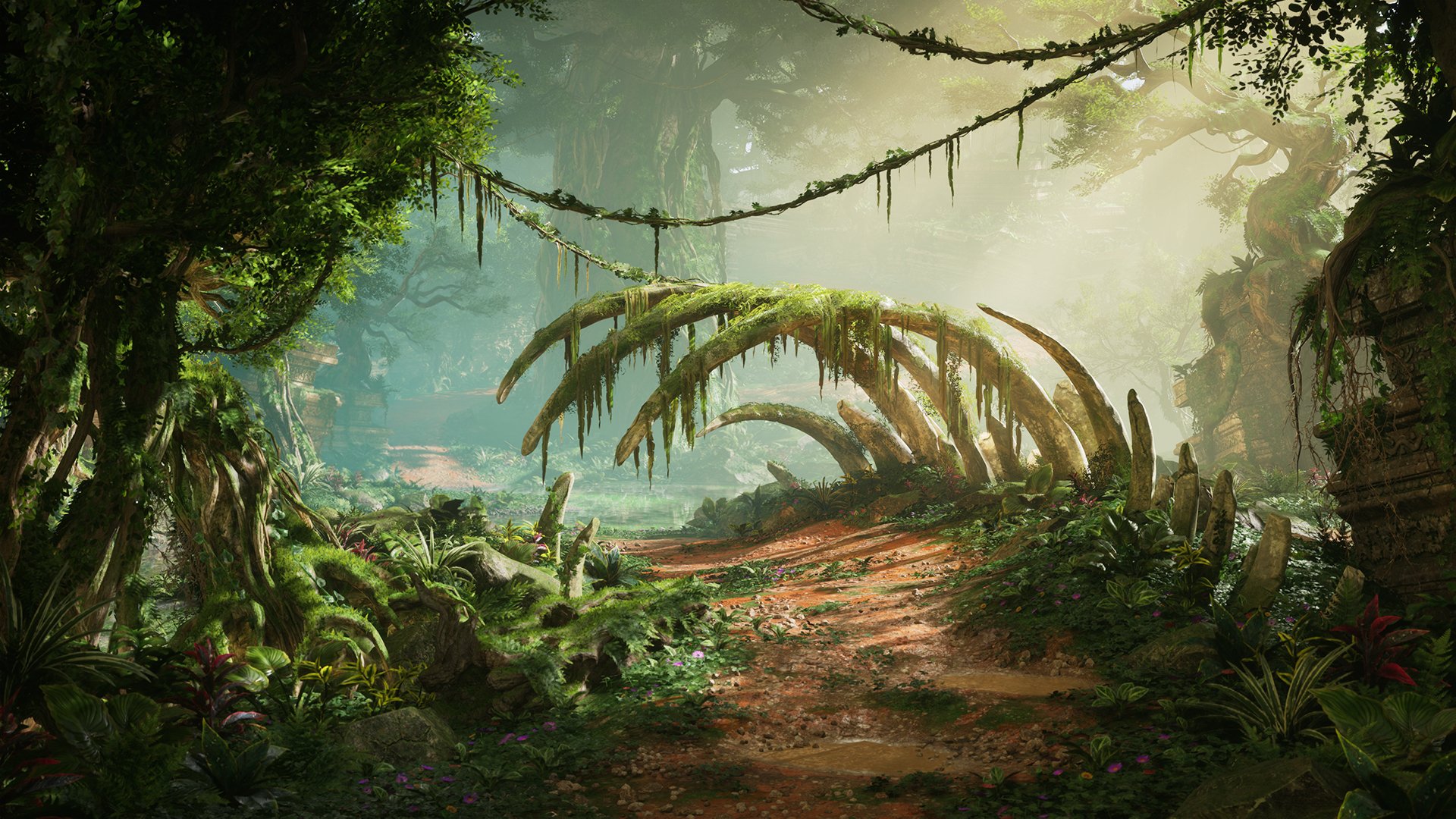This is a detailed computer-generated color illustration depicting a dense and dark jungle. The scene is dominated by towering trees with giant trunks and extensive root systems, their thick canopies allowing only small patches of sunlight to filter through. The central dirt path, a rich dark brown or red clay, appears recently rained on, with tiny pools of water at the forefront. The path curves toward the center, accompanied on each side by lush grasses and vegetation, and eventually leads into the depths of the jungle.

The most striking feature is an archway formed by the immense moss-covered ribcage of an unidentified, presumably massive animal, hinting at the ancient and mysterious nature of the jungle. Vines, heavy with dripping vegetation, swing from tree to tree, adding to the sense of wild, untamed beauty. To the far right, a crumbling stone pedestal supports a tree with gnarled branches reaching leftwards. In the center background stands a gigantic tree, anchoring the composition and enhancing the scene's enchanted atmosphere. The blurred background nonetheless reveals additional greenery and trees along the pathway, emphasizing the dense and all-encompassing nature of the jungle.